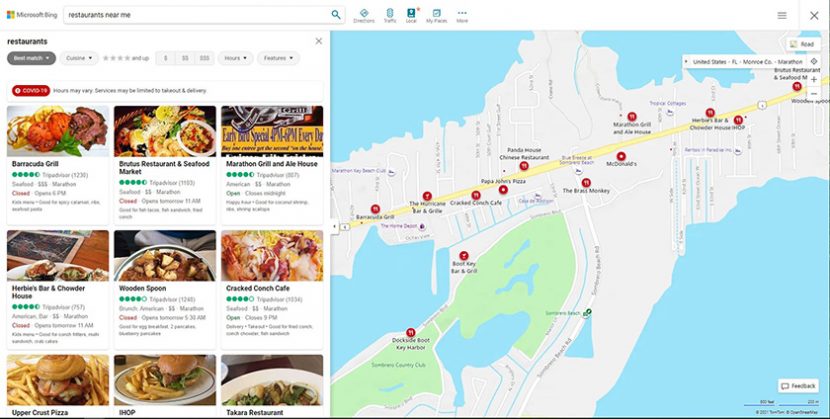This image depicts a search results page from Bing, displaying local restaurant listings. At the very top of the page, you see the Bing logo accompanied by the Microsoft logo on the left side. Below the search bar, the word "restaurants" is highlighted in bold. Beneath it, within a gray box, the term "Best Match" is featured, followed by the word "cuisine" and a star rating with star symbols to the right.

At the very top of the listings, a COVID-19 disclaimer warns that hours may vary, and services might be limited to takeout and delivery. Following this disclaimer, a list of nine restaurants is presented.

1. **Barracuda Grill**: The first restaurant listed.
2. **Brewer's Restaurant & Seafood Market**: Adjacent to Barracuda Grill on the right.
3. **Marathon Grill & Owl House**: Listed next to Brewer's Restaurant & Seafood Market.
4. **Herbie's Bar & Chowder House**: Appears below Barracuda Grill on the left.
5. **Wooden Spoon**: Right next to Herbie's Bar & Chowder House.
6. **Craft Conch Cafe**: Located to the right of Wooden Spoon.
7. **Upper Crust Pizza**: This entry is on the left of the bottom row.
8. **IHOP**: Listed next to Upper Crust Pizza.
9. **Taqueria Restaurant**: The final listing on the right side.

The upper segment features visible ratings and brief descriptions for each restaurant. However, the bottom portion of the listings for the last three restaurants is partially obscured, making it difficult to see the full details.